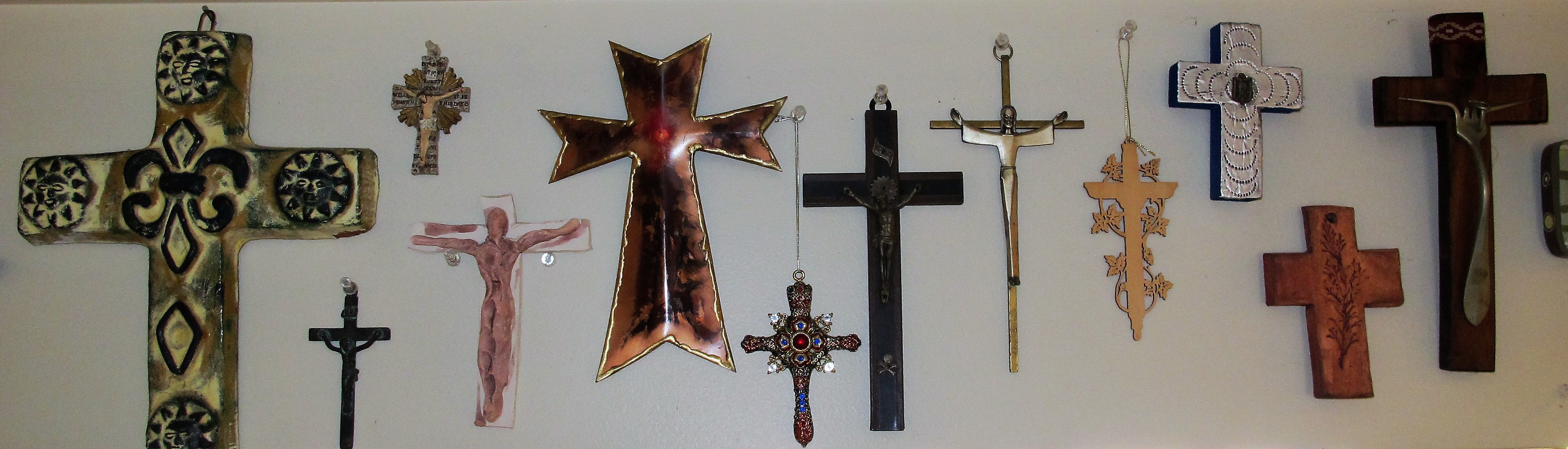This photograph showcases a diverse collection of crosses and crucifixes mounted on an off-white wall. The subdued lighting highlights the varied materials and designs, emphasizing the rich tapestry of each piece's significance. Among the array, there are simple wooden crosses next to intricate metal ones. Notable designs include a black marble cross with white veining, a modern silver crucifix towards the center, and a jewel-encrusted silver cross with red gemstones. Historical and symbolic pieces are also present, such as a Flor de León cross. There's a gold cross with elaborate patterns of diamonds, circles, and lines, and a light pink crucifix depicting Jesus' body. The assortment also features brass, clay, and light gold crosses, each distinct in its craftsmanship. This detailed display underscores the universal and historical symbolism of the cross.